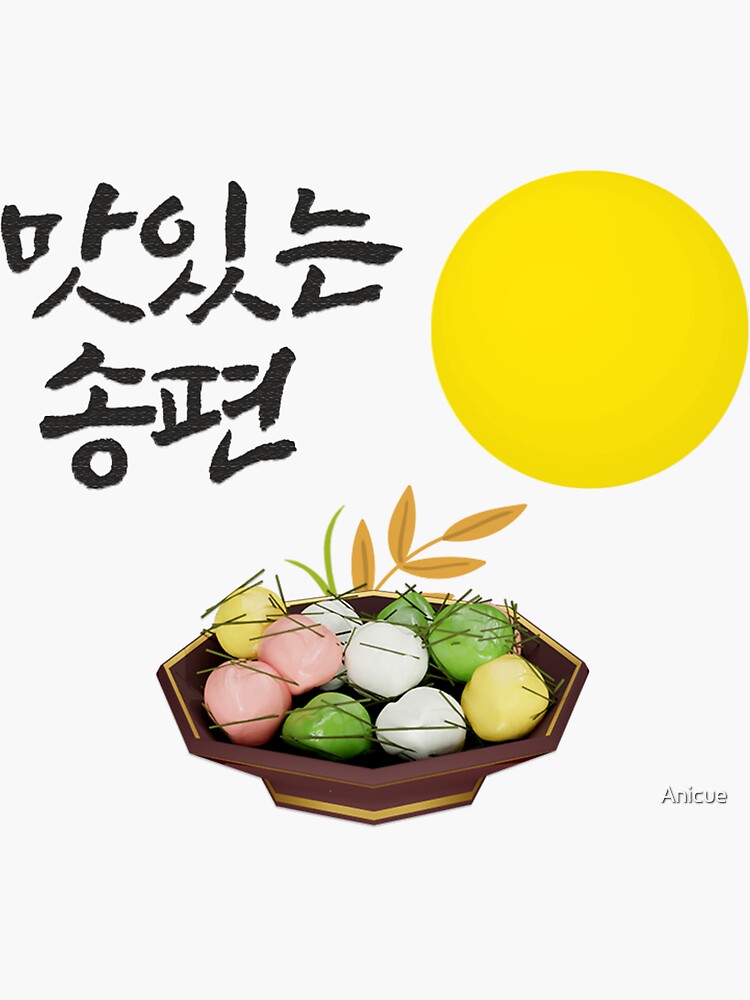This image is an advertisement featuring Japanese writing at the top left corner, though the exact meaning is unclear. The main focus of the image is a cartoonish depiction of a small bowl or platter filled with round, multicolored items. The items in the bowl are primarily pink, yellow, white, and green, resembling Easter eggs, candies, or possibly pieces of fish or tofu. The food in the bowl appears to be drizzled with a black sauce. Behind the bowl, there's a yellow sun icon against a white background, accompanied by drawings of brown leaves and green grass, adding a whimsical touch to the overall composition. The advertisement is likely produced by Sony, indicated by the labeling.